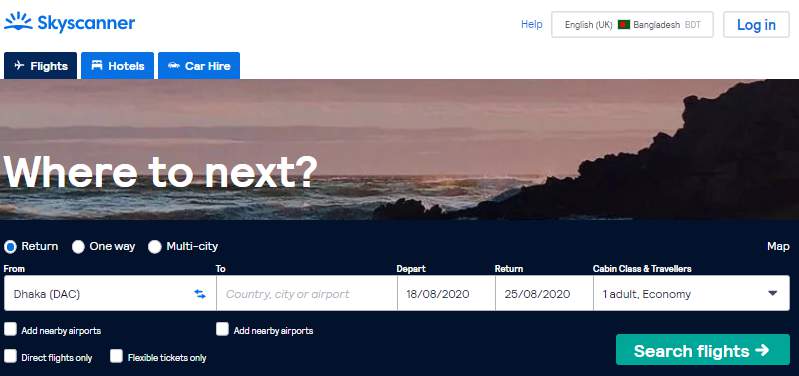The image is a detailed screenshot taken from the flight booking website, Skyscanner. The layout of the image is horizontal and more elongated, with approximate proportions of 30 to 70. 

In the top left corner, the Skyscanner brand is prominently displayed in blue text alongside a logo depicting a blue sun rising over a horizon. Moving to the right side of the header, there are options for help, language selection (showing "English UK" and "Bangladesh" with the corresponding flag), and a login button.

On the left side of the screen, three tabs are visible: "Flights" (highlighted with a navy blue background), "Hotels," and "Car Hire" (both in royal blue). 

Below this section, a large horizontal image spans the width of the screen. This background features a scene of a dark hill facing a sea under a pink sky, suggesting an early evening or late sunset ambiance. Overlaid on this image are the words "Where to next?" in white letters.

Immediately below this banner, flight search options are prominently displayed. These options include:
- "Return" (which is selected),
- "One-way," 
- "Multi-city."

Further down, search parameters are filled in as follows:
- Departure city: Dhaka (DAC),
- Destination: Country, city, or airport,
- Departure date: 18/08/2020,
- Return date: 25/08/2020,
- Cabin class and travelers: One adult, economy.